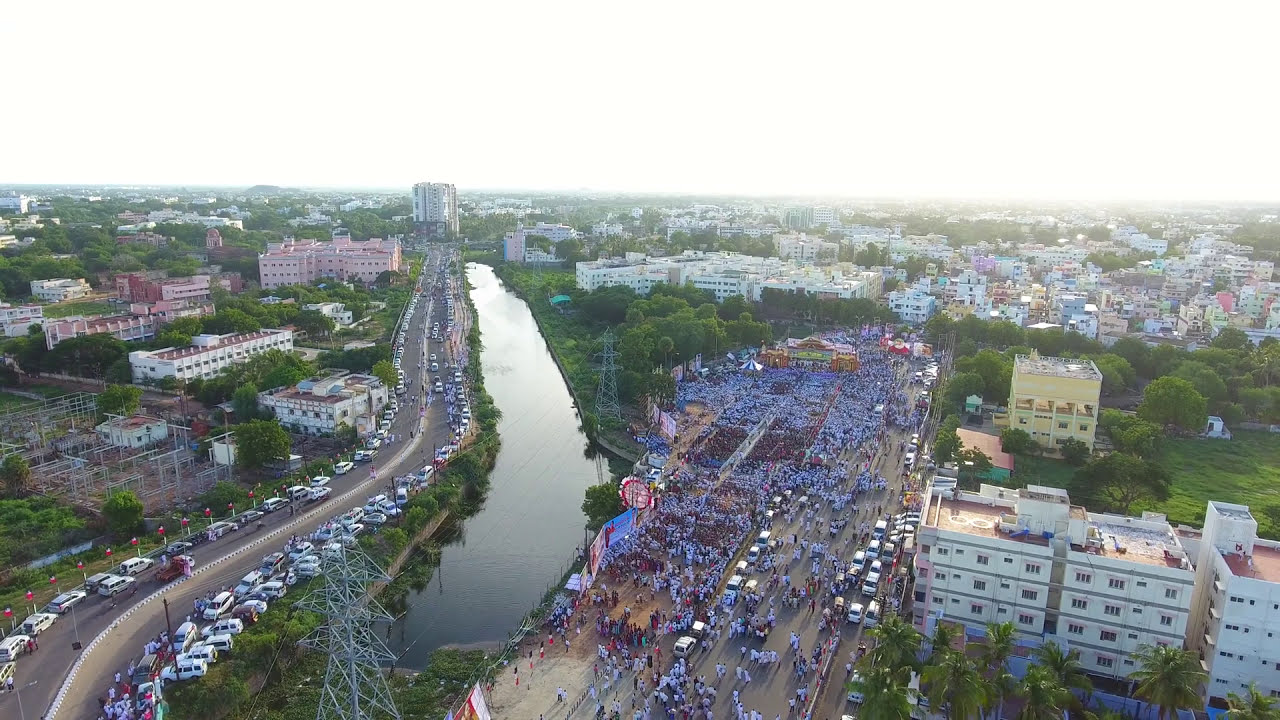This aerial color photograph provides a detailed and vibrant view of a bustling urban scene. Centrally featured is a narrow body of water, possibly a river or a pond, with roads running parallel on both sides. The left side of the water is lined with numerous parked cars and additional vehicles in motion. The road on the right side of the water, a large boulevard, is densely populated with thousands of people, suggesting a significant event or procession is taking place. 

The urban landscape is dotted with a variety of buildings, ranging in color from pink and yellow to light purple, turquoise, and green, with notable structures including several multi-story, blocky white apartment buildings. The foreground and midground reveal this vibrant activity, while the background indicates a densely built cityscape surrounded by greenery. Additionally, electricity towers are visible near the water body, adding to the urban infrastructure. The sky above is a solid white, creating a stark contrast with the colorful, dynamic cityscape below.